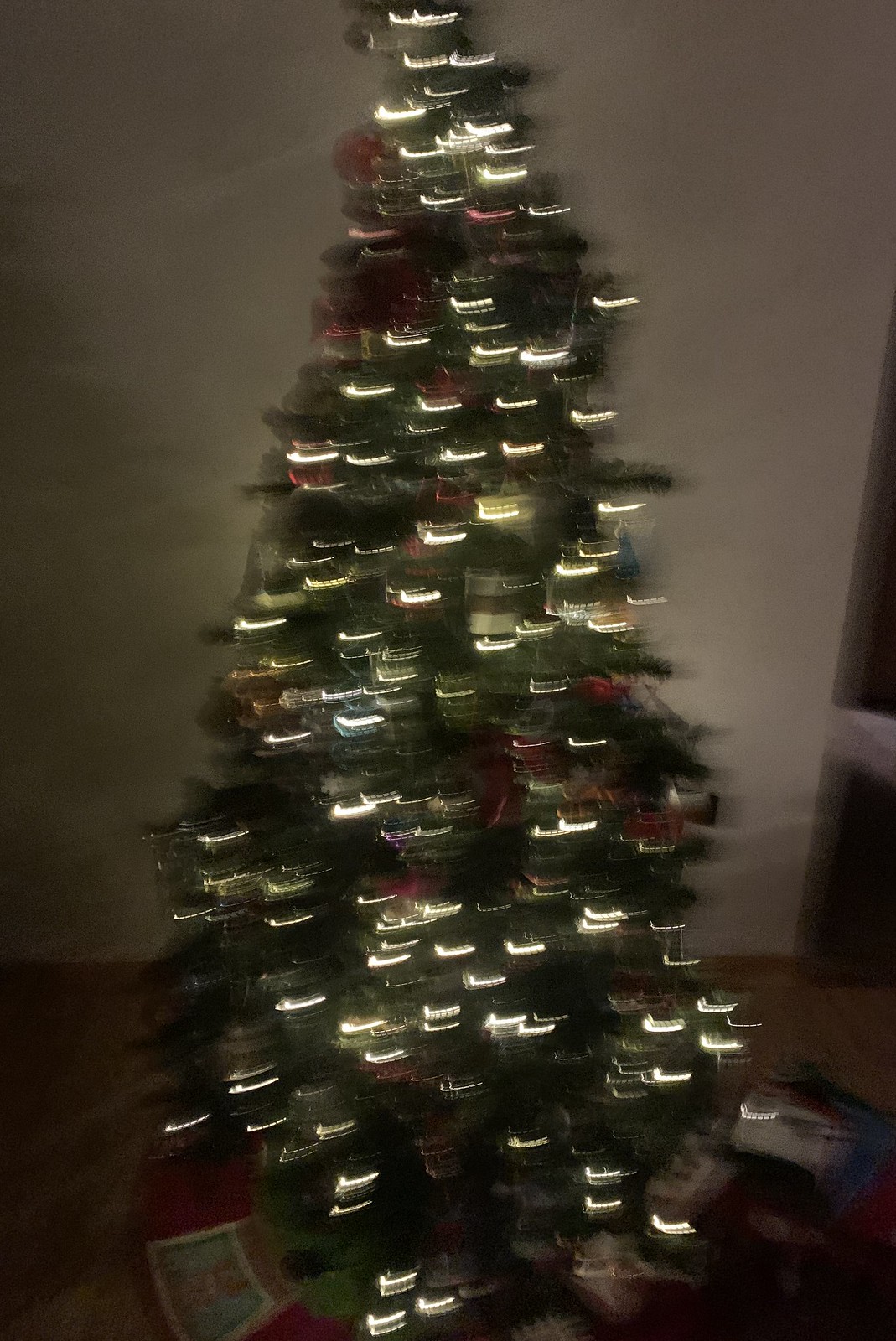Vertical image of a Christmas tree, captured in low light against a white wall. Due to the long exposure and movement of the camera from left to right, the white lights adorning the tree appear as small hockey sticks or elongated lines with tail hooks. Scattered among the lights are visible red and gold ornaments, adding festive color to the scene. The tree itself seems to be a short-needled fir or cedar type. Dark, shadowy presents are discernible underneath the tree, contributing to the dim and evocative interior atmosphere of the photograph.